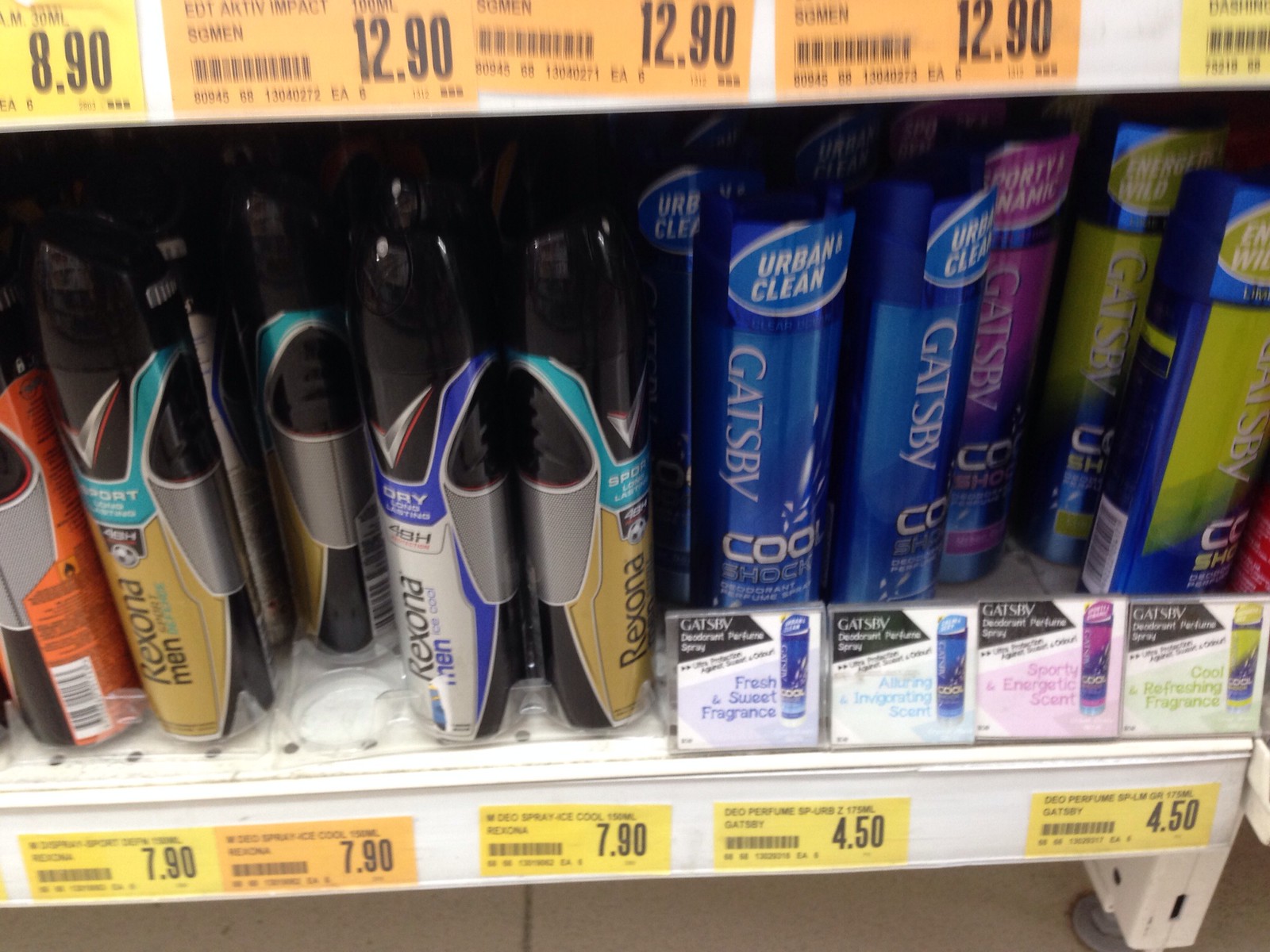This photograph is a close-up, color snapshot of a cream-colored metal grocery shelf in a store, lined with aerosol cans of deodorant from two different brands. The shelf, which runs horizontally from left to right, features yellow and orange price tags with barcodes along the top and bottom edges. The left side of the shelf displays various colored cans labeled "Rexona for Men," in shades of gray, orange, gold, light blue, and dark blue. In the center of the image, the Rexona cans transition to "Gatsby" branded deodorants on the right, featuring cans in dark blue, pink, and green. The Gatsby cans have additional tags indicating their "Urban Clean" scent, and display prices ranging from 4.50 to 7.90 euros. The entire arrangement is slightly elevated off the floor, emphasizing the neat rows of metallic, aerosol products neatly aligned on the shelf.